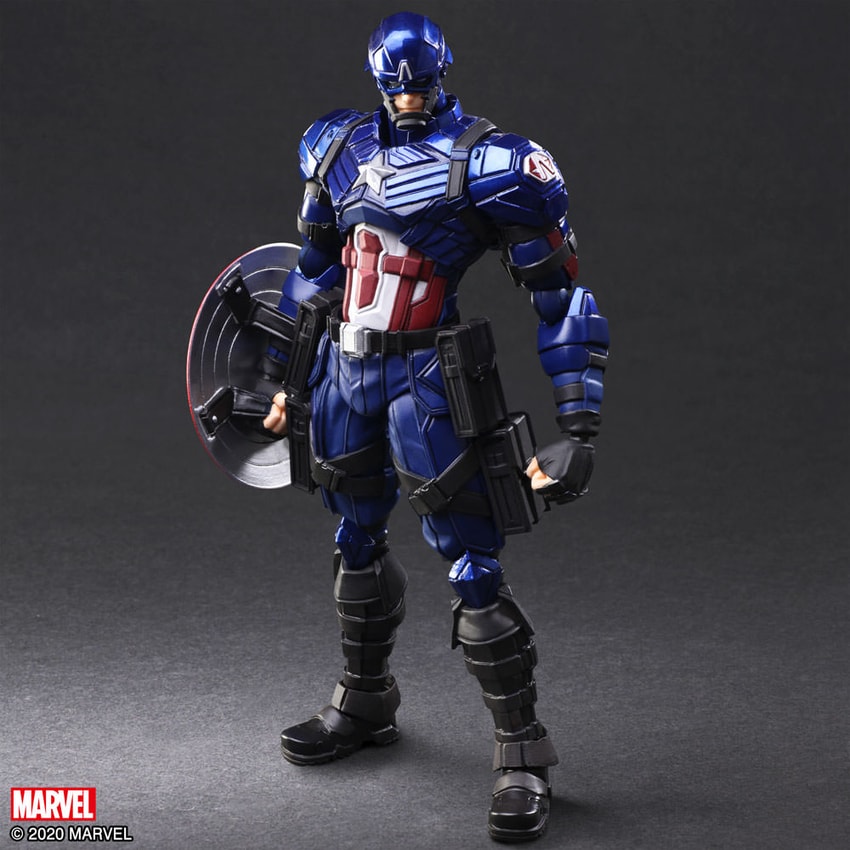The image showcases an action figure of Captain America, adorned in his iconic blue suit and helmet with black lines, accented by a prominent white star on the chest. His suit features a red and white pattern at the torso, embodying the traditional American colors. Captain America is depicted wearing black knee-high boots and a face mask with the letter 'A' on his forehead. He wields his unmistakable shield on his right arm, with the metal back and red border visible. The figurine also features compartments hanging from his hips, and clenched fists add to his ready-for-action stance. At the bottom left corner of the image, the Marvel logo and the copyright "2020 Marvel" are clearly visible. The background is composed of various shades of gray, contributing to a darker, more intense atmosphere.